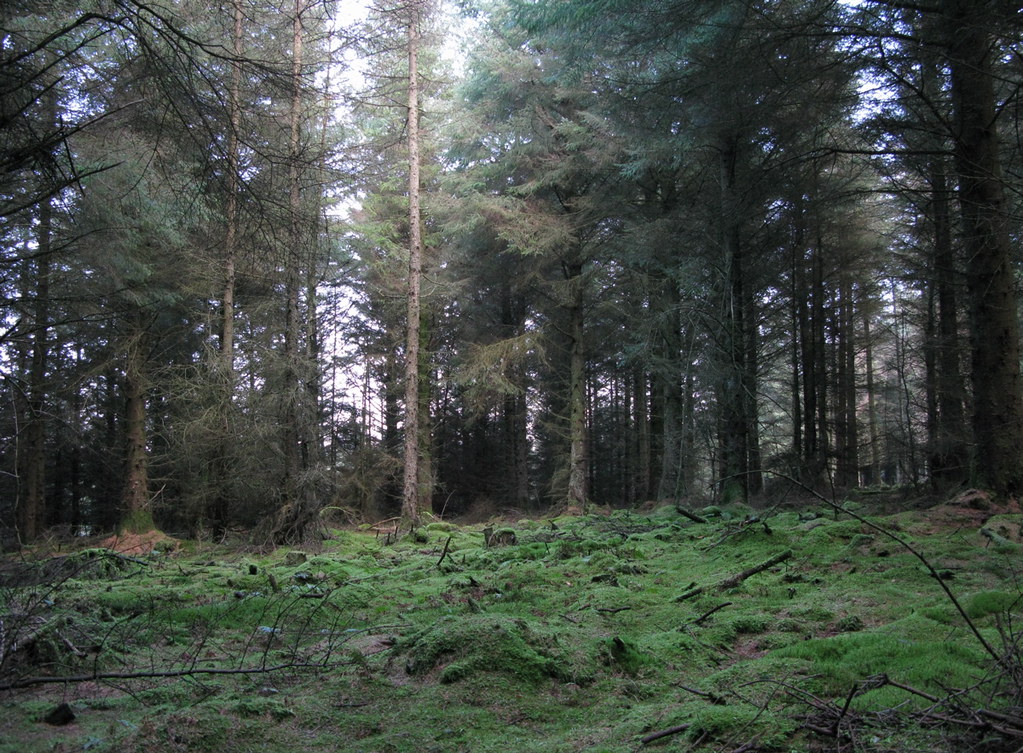This is a horizontally aligned rectangular image taken outdoors in a heavily wooded forest area. The background is dominated by very tall, narrow tree trunks, likely pine or evergreen trees, with feathery green leaves that block out much of the sky. However, patches of bright white and blue sky are visible through the dense canopy. The foreground reveals a forest floor covered in green moss, grass, and various green plants, interspersed with small mounds of dirt and scattered with numerous broken branches and twigs. The floor appears flat but has small undulating hills of greenery. Bare branches and twigs punctuate the scene, with some lying on the ground and others sticking out, suggesting an area that may have been cleared before starting to regrow its vegetation. The scene exudes a sense of tranquility and scenery, capturing the majestic essence of this lush forested area.